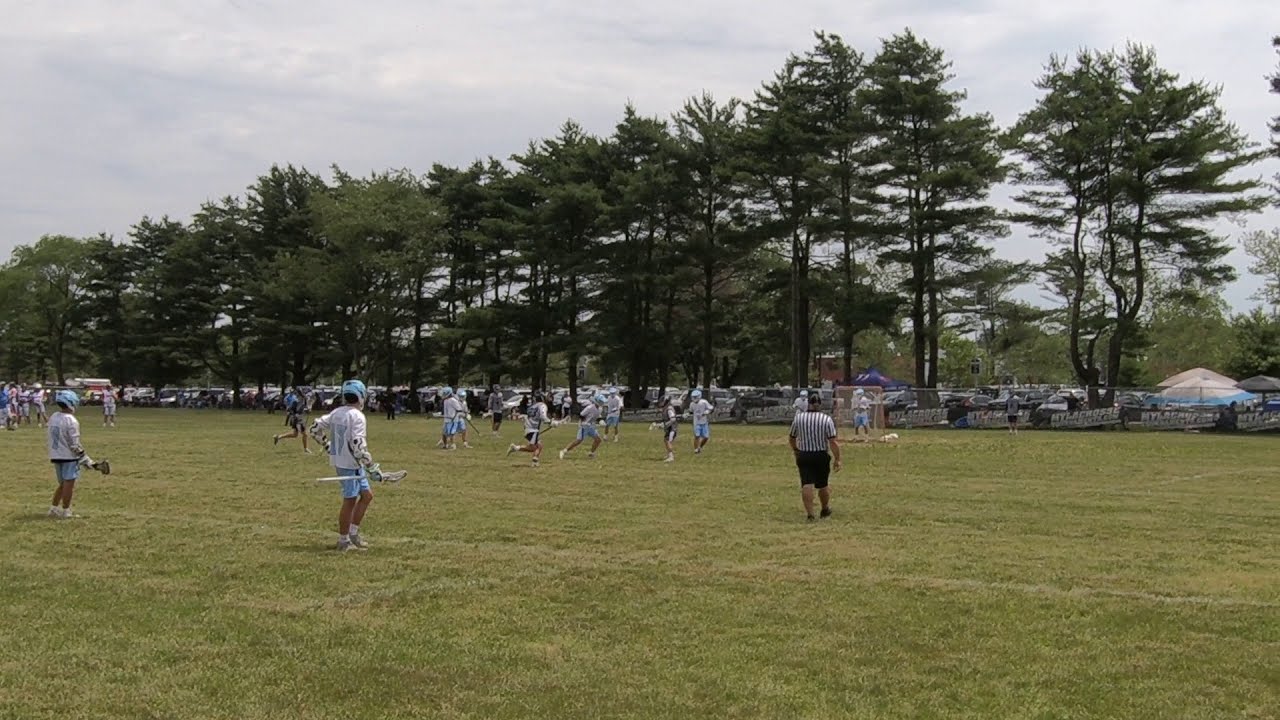This detailed photograph captures an outdoor lacrosse game in action on a lush, green sports field. The field is flanked by tall deciduous and large pine trees, with a row of parked vehicles and a fence adorned with various banners and posters visible in the background. Above, a blue sky dotted with white clouds adds to the scene's vibrancy.

Two teams are engaged in the game: one team wearing white shirts with blue shorts and blue helmets, and the other donning white shirts with black shorts and black helmets. The players are actively involved, seen wielding lacrosse sticks as they maneuver around the field. The action is concentrated near the goal areas, with some players positioned at the far end, even though the goal itself is not visible. 

A referee, distinguishable in his black and white vertically striped shirt and black shorts, is seen walking towards the players, adding an official touch to the game. In the distance, other people are observed lining the fence area, some seated under areas that might be umbrellas or shaded spots, watching the game unfold. The lively tableau exudes the energy and competitiveness of a daytime lacrosse match.